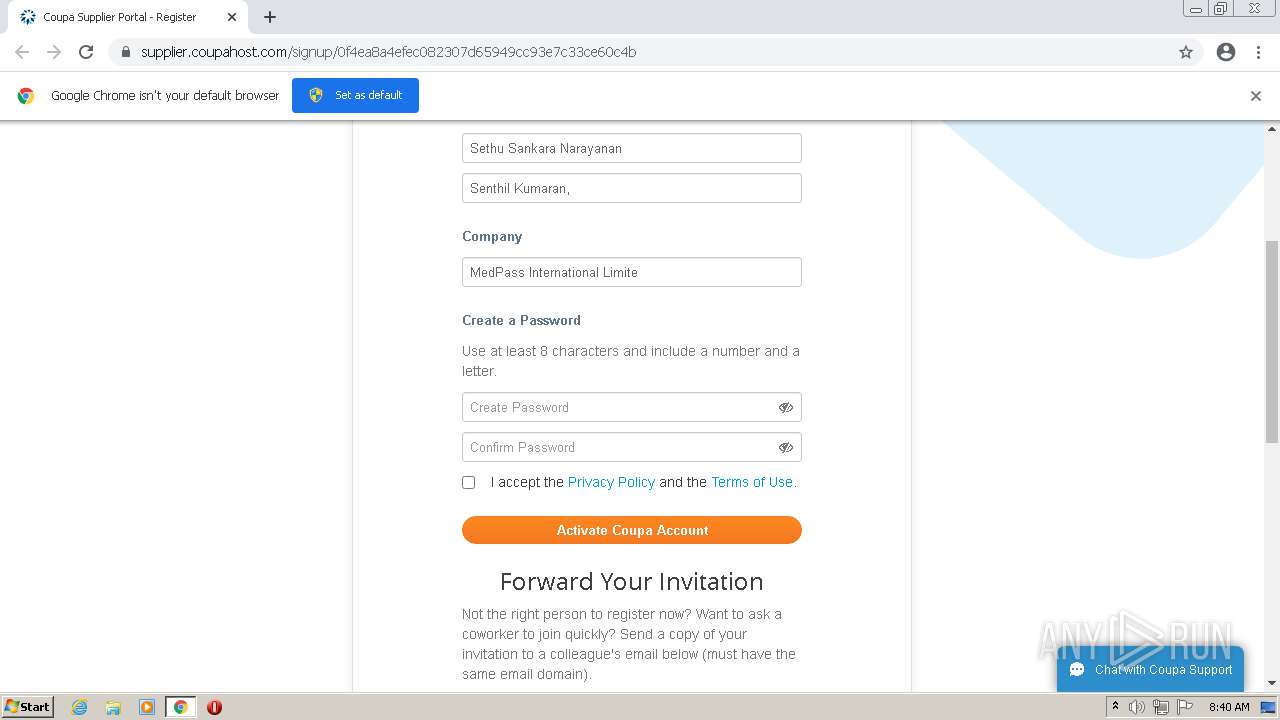In this color screenshot, captured in landscape format, we see a computer screen displaying a browser window, specifically Google Chrome. The user is on the "Koopa Supplier Portal Register" webpage, accessible via the URL: supplier.koopahost.com/sign-up, followed by several alphanumeric characters. A notification at the top indicates that Google Chrome is not the default browser, with an option to set it as default available.

The visible portion of the webpage shows a registration form partially filled out. The user's name, "Sethu Sankara Narayanan," and company, "Medpass International Limited," are inputted in the respective fields. Below, a section prompts the user to create a password, advising them to use at least eight characters, including both a number and a letter. This area is currently blank, awaiting input.

Additionally, the form requires the user to accept the privacy policy and terms of use, which haven't been checked yet. Once these fields are completed, the user can click the prominent orange "Activate Koopa Account" button at the very bottom of the form.